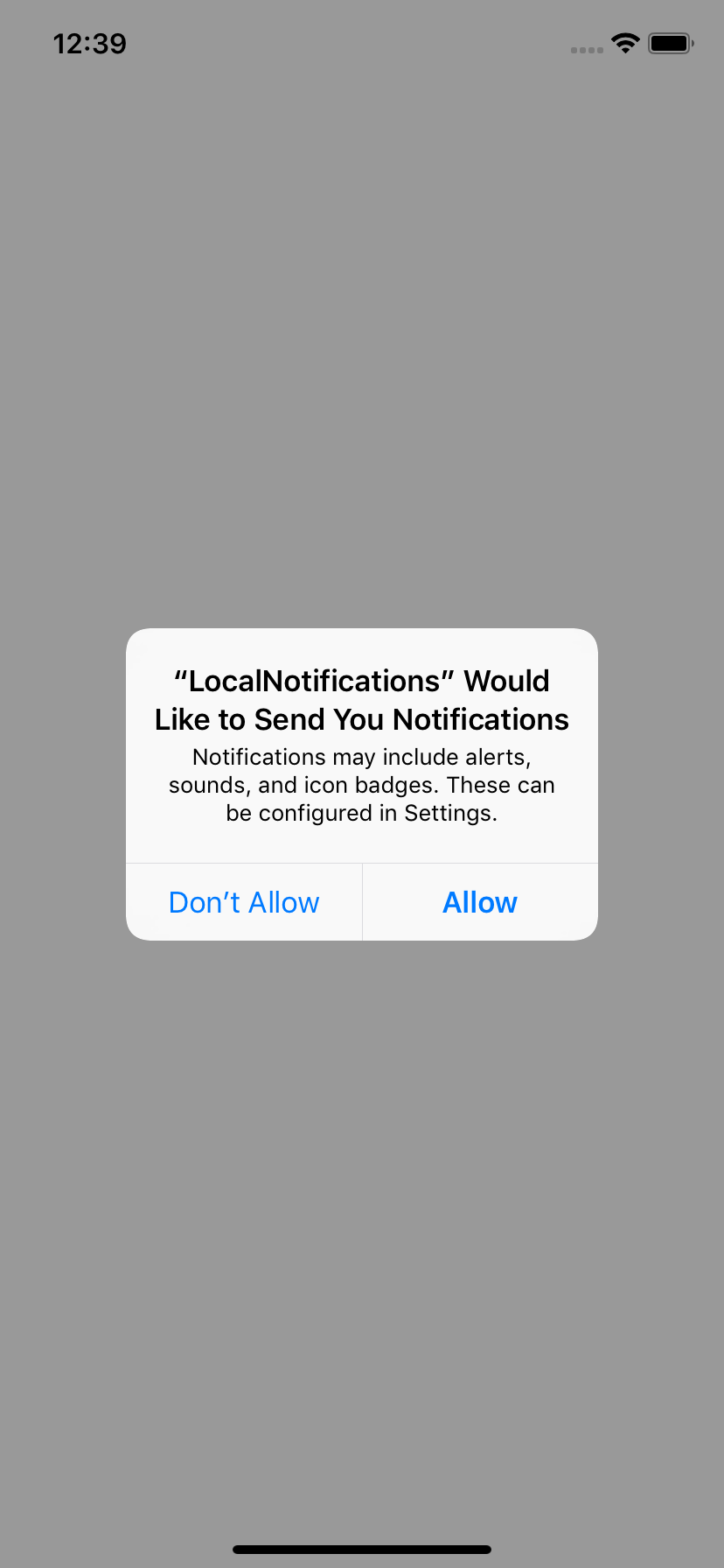This screenshot captures a notification alert from an Apple application on an iPhone, highlighted against a blurred, grayscale background of the user interface. The top left corner of the screen displays the current time in black text, showing "12:39". To the right, there is an icon for cellular signal strength, which currently shows no bars, indicating no reception. Continuing to the right, the Wi-Fi icon is fully filled, indicating a strong connection with three out of three bars. Adjacent to the Wi-Fi icon, the battery percentage icon shows a full charge at 100%.

Dominating the center of the screen is a white rectangular alert box requesting permission for notifications. At the top of the rectangle, in bold text, the header reads "(Local Notifications)". Below this header, the main message in quotations states, "Local Notifications would like to send you notifications." Following this, a subtitle explains, "Notifications may include alerts, sounds, and icon badges. These can be configured in settings."

At the bottom of the alert box, there are two options presented in blue text. The button on the left reads "Don't Allow," and the button on the right reads "Allow." This neatly structured notification prompts the user to make a decision regarding the app's permission to send notifications.